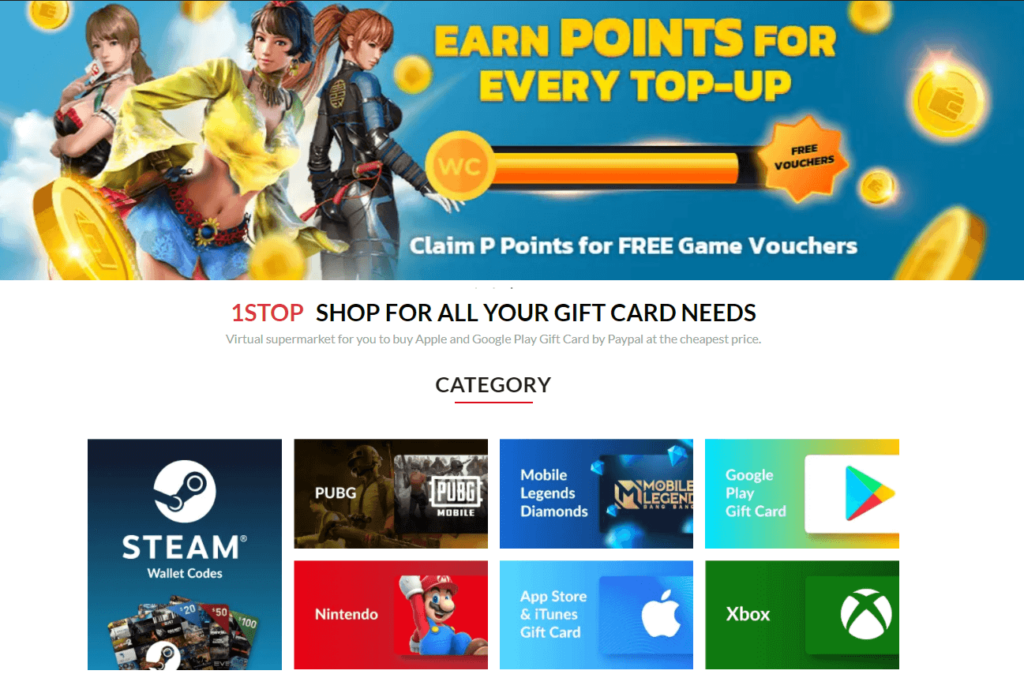The image depicts a vibrant landing page with a prominent banner at the top featuring digitally generated female characters, who appear to be Asian, dressed in various elaborate outfits. 

On the left, a character with brown hair tied in a ponytail and extending to shoulder length holds a white card adorned with a red heart. She is dressed in a black dress with frills accentuating the top of her chest.

At the center stands another character, adorned in a short, golden-yellow Victorian-era blouse with parachute-like sleeves. She sports a gold necklace, a short brown hairstyle with a red flower, and a blue skirt with a red belt featuring a gold buckle. Her left hand rests confidently on her hip.

To the back stands a character with long hair (tied in a ponytail) that would reach past the middle of her back if let down. She has short bangs and is clad in a two-piece leather suit - black on top and blue below. Her gear appears tactical, and she wields a sword with a red hilt. Beside her, digital orange coins are scattered, indicating some form of reward system.

On the right side of the banner, text reads: "Earn points for every top-up," followed by a coin graphic with "WC" nearly filling the coin. Below it, promotional text in dark blue proclaims, "Claim points for free game vouchers," with highlighted details beneath: "One stop, SHOP for all your gift card needs," and further descriptive text indicating a "virtual supermarket" offering Apple and Google gift cards via PayPal at the best prices.

Further down, various gift cards are categorized:
- **Steam cards:** Nominal values of $20 (blue), $50 (red), and $100 (green).
- **PUBG (PlayerUnknown’s Battlegrounds):** Details provided in a black background.
- **Mobile Legends Diamonds:** Displayed on a blue background.
- **Google Play gift card:** Featured on a teal, orange, and yellow background with a Google Play logo.

The listing continues with a Nintendo section, indicated by Mario in his traditional red and blue costume against a red backdrop, and a white circle enclosing the word "Nintendo."

Lastly, the section showcases:
- **Apple Store and iTunes gift cards:** A blue card with a white apple logo.
- **Xbox gift card:** Depicting the Xbox logo, a circle with a green X.

This detailed narrative highlights the array of items and offers available on the digital marketplace landing page.